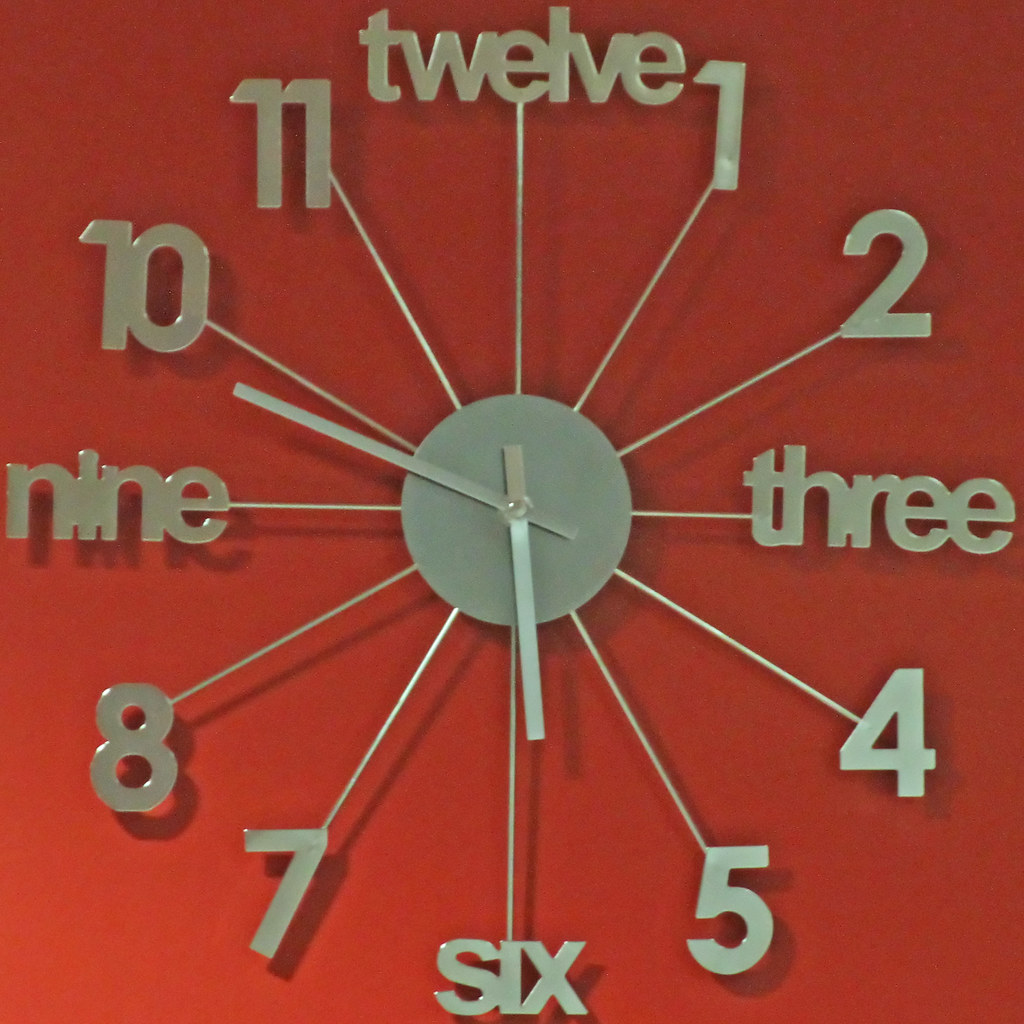This photograph features a unique wall clock with an orange background, though it could be an arrangement of metal numbers and hands directly affixed to the orange-painted wall. The clock itself is composed of metal elements. Notably, the 12, 3, 6, and 9 positions are denoted by lowercase words ("twelve," "three," "six," and "nine"), while the remaining hours—1, 2, 4, 5, 7, 8, 10, and 11—are represented by metal numerals. Each numeral and word is connected to a central metal circle by slender rods. This central hub houses the clock's silver-colored hour and minute hands, which are pointing to approximately 5:49.